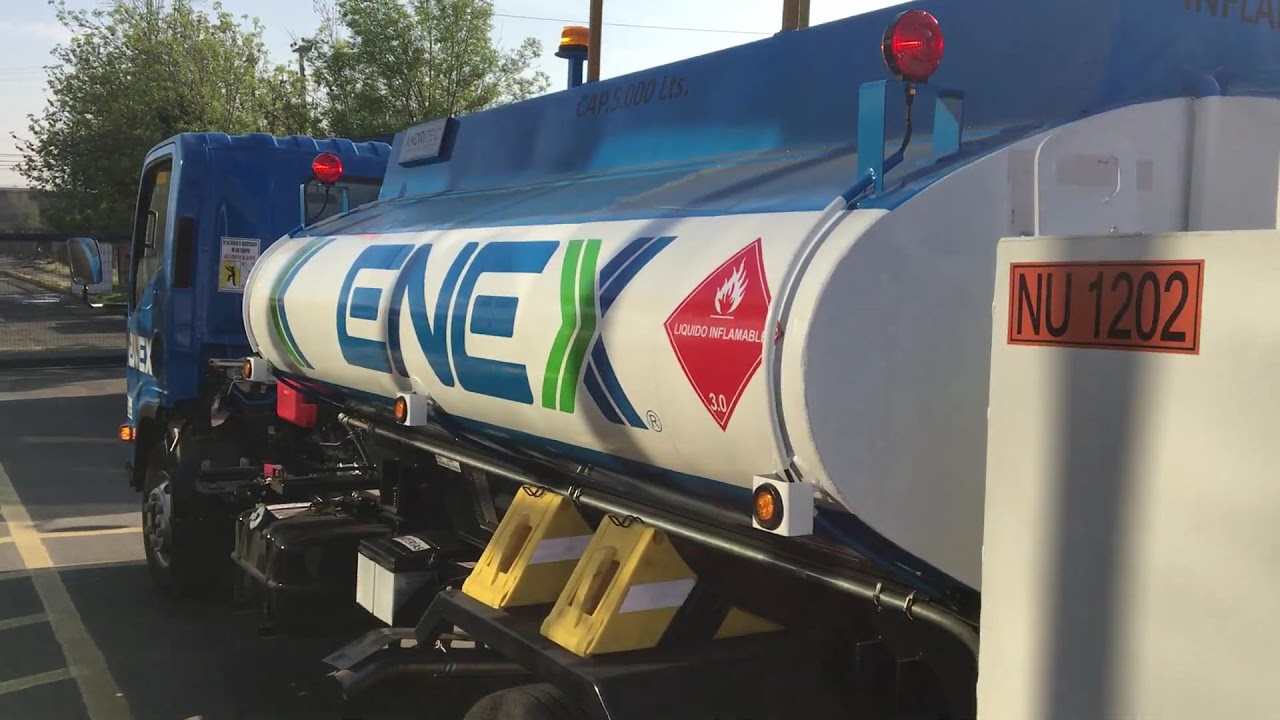The image features a side view of a tanker truck, most likely an oil or petroleum transporter, positioned on a roadway with a visible pedestrian walkway. The truck's cab is blue, and the main tanker, which is blue and white with green accents, prominently displays the letters "ENEX." The "E N E" is in blue, while the "X" combines green and blue hues. Additionally, there is clearly marked text reading "Liquido Inflammable" in white against a bold red background, accompanied by a red hazard sign with the number "3.0" and a fire symbol.

Further details reveal an orange box with "NU-1202" on the tanker, and above it, the text "CAP. 5,000 liters" is visible. The tanker is secured by black tires, with two yellow wedges positioned underneath to prevent rolling. The scene also includes the black asphalt road with yellow stripes, green trees, and a visible electrical line in the background.